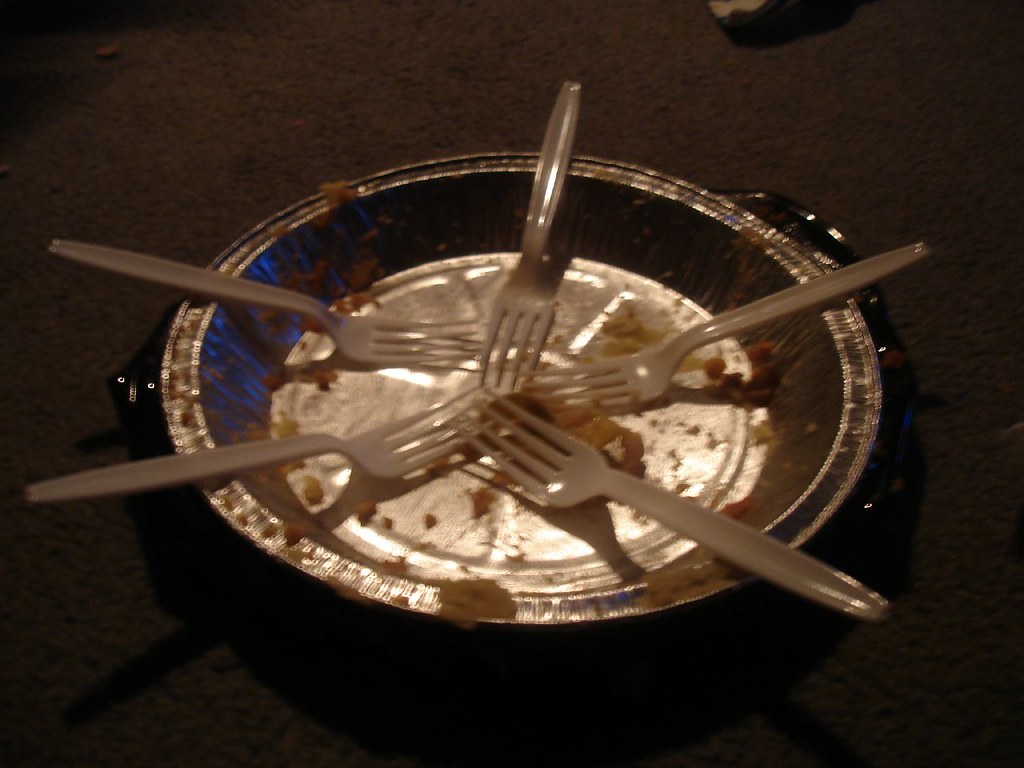The photograph captures a dimly lit scene focusing on an aluminum pie tin, nestled within a glass container and sitting on a nondescript, dark surface, the specifics of which remain indiscernible. The aluminum pie tin, lightweight and characterized by its crimped edges, is empty except for a few scattered crumbs of crust clinging to the bottom and edges. Arranged in a star-like configuration, five white plastic forks are evenly spaced within the pie tin, their clean handles extending outward from the center, indicating they were likely used to consume the now-absent pie. The background of the image is too dark to reveal any additional details, contributing to the overall lack of clarity in the photograph.